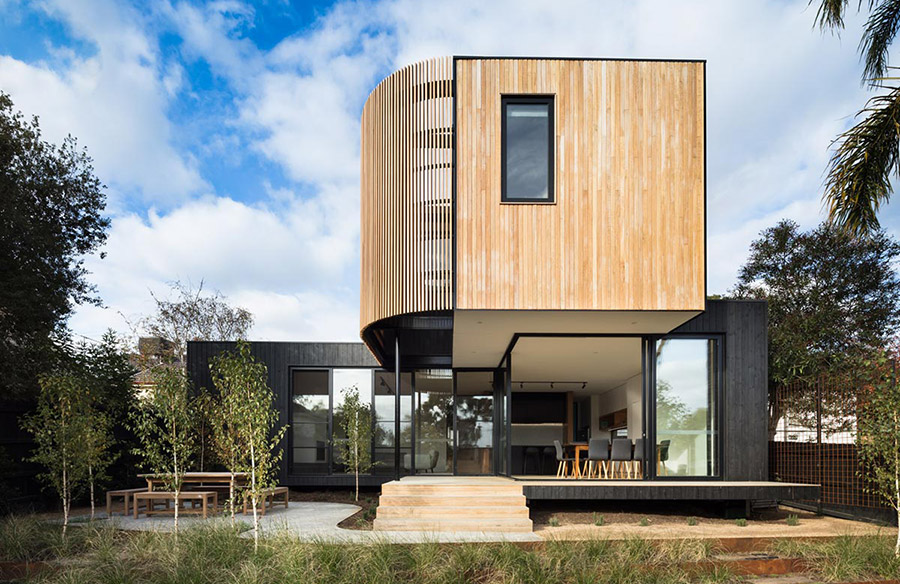The image is a detailed 3D color illustration, likely created using an application like SketchUp, showcasing a strikingly modern, two-story structure nestled within a natural setting. The building features a unique design, characterized by a lower level with an almost L-shaped form, made predominantly of glass and wood. The large glass windows offer an unobstructed view inside, revealing a dining table surrounded by black leather chairs. 

The upper floor is a cantilevered square structure, clad in light wood paneling, with a smaller vertical window on the front. The left side of the upper level has a distinctive curved, accordion-like section with horizontal boards that are semi-transparent, allowing glimpses of the windows behind. 

The house is set in a verdant area with long grass, bordered by both smaller, newly planted trees and larger, mature trees. A beautifully blue sky with scattered clouds forms the backdrop, suggesting a warm climate, further hinted by the possible presence of palm trees in the top right corner.

The front of the house features a paved area and a wooden porch with steps leading up to the entrance. The entire scene exudes the ambiance of a luxurious, summer day in a sophisticated yet natural environment.